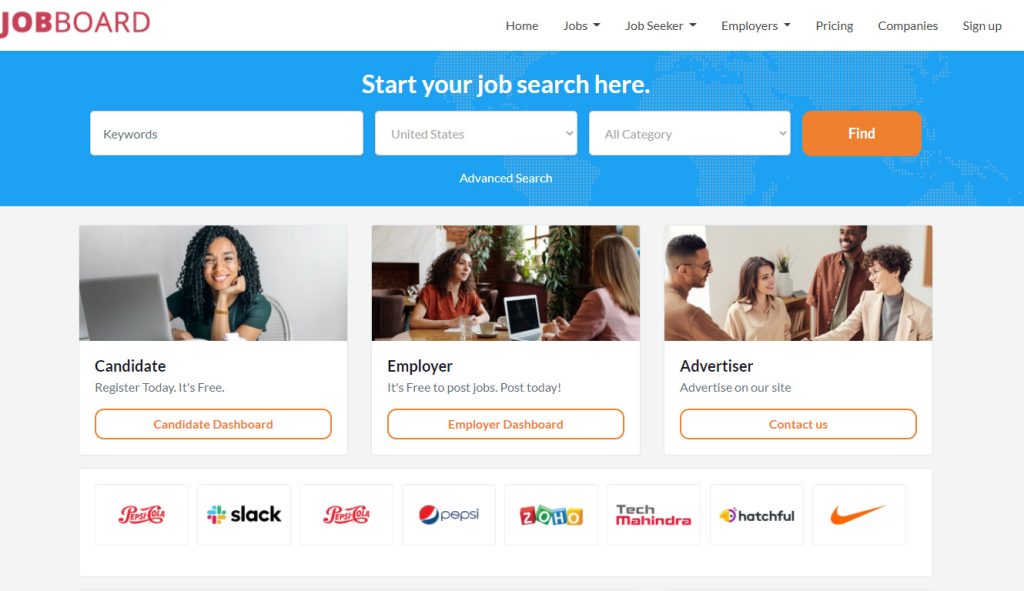The image showcases the Job Board website interface. In the top-left corner, the website name "Job Board" is prominently displayed, with "Job" in bold red font and "Board" slightly less bold but still in red. Centrally placed on a white banner at the top are navigation links: Home, Jobs, Job Seeker, Employers, Pricing, Companies, and Sign Up. The options for Jobs, Job Seeker, and Employers feature drop-down arrows indicating additional sub-menu items.

Beneath this white navigation banner is a blue banner with the bolded white text that reads "Start Your Job Search Here." Directly below this are three white rectangular input fields for keyword search and location filtering; the second and third fields specifically read "United States" and "All Categories," each with their own drop-down arrows. An orange rectangular button marked "Find" with white font is situated next to these input fields. Below this search section is the link text "Advanced Search."

Further down, the page is sectioned into three distinct media image categories labeled Candidate, Employer, and Advertiser. The Candidate section features an image of a young Black woman in her 20s, wearing glasses and smiling with her hand resting under her chin. The Employer section includes a picture of two individuals sitting across from each other at a desk. The Advertiser section shows a group of individuals. Each image has corresponding action buttons below them.

At the very bottom of the image, several recognizable corporate logos are displayed, including those of Pepsi Cola, Slack, Tech Mahindra, and Nike.